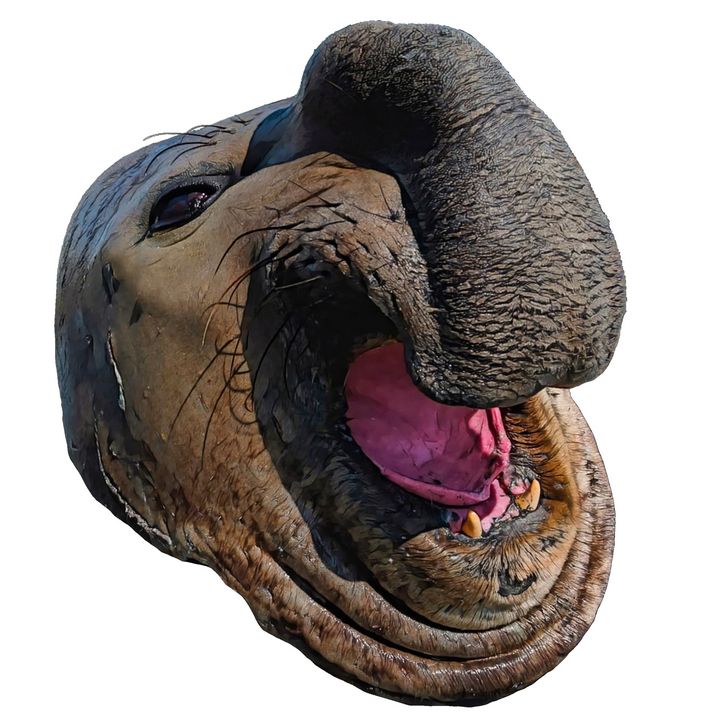The image showcases a detailed and unusual sculpture, possibly crafted from clay or papier-mâché, depicting a fantastical creature resembling an elephant. The head features a large, intricately textured trunk folded up against the face, emphasizing the bizarre nature of the piece. The creature's open mouth reveals a reddish-pink tongue, curled upwards, and noticeable yellow bottom fang-like teeth. One black eye is visible, adding to the lifelike yet eerie appearance. The lighting highlights the lower part of the mouth, chin, and the left cheek, enhancing the textured details. Whiskers or hair-like structures sprout from various parts of the head, including around the eye and on top, contributing to its strange, almost surreal quality. The overall color palette leans towards brown with reddish accents in the mouth area, making the sculpture both mesmerizing and unsettling.